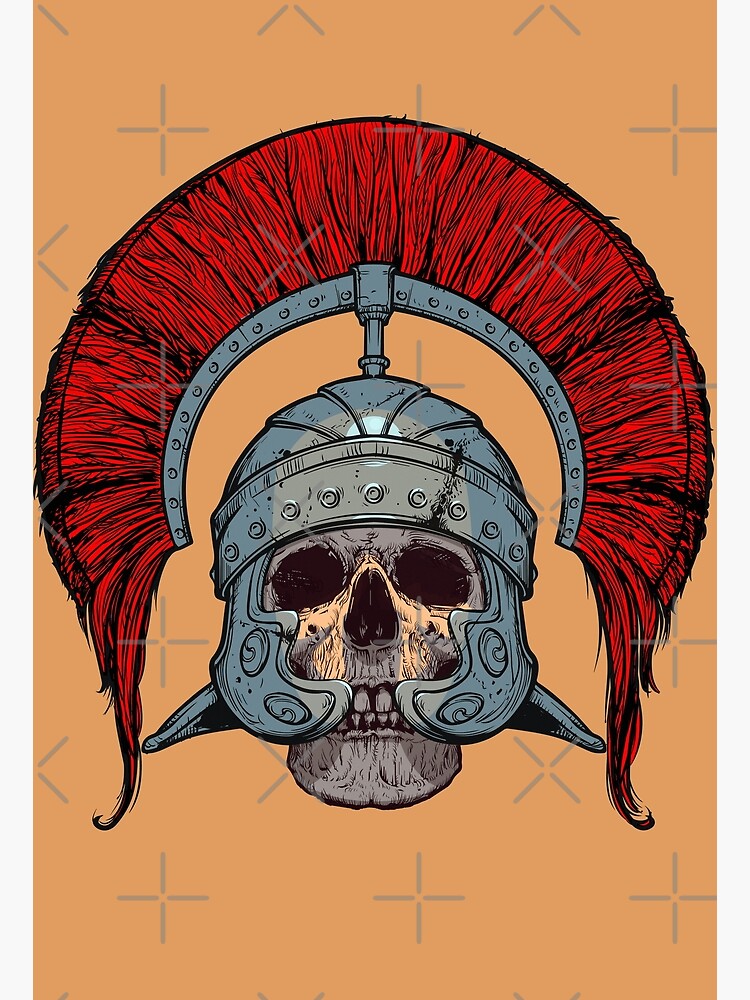The image is a detailed digital artwork featuring a prominently centered skull adorned with an ancient Roman helmet. The background is a vivid orange, crisscrossed with numerous small silver star-like and cross shapes, which give it an intricate, almost tapestry-like texture. The skull's helmet is reminiscent of those used by Roman soldiers, with a pronounced red brush resembling fanned feathers or horsehair on the crest, shaped into a semi-circle that forms a frowning arch above the skull. This red crest is supported by a metal band at its base, attached to the main helmet structure via a small rod. The helmet itself envelops the skull, extending down over the cheeks in crescent moon shapes and covering the forehead. It also protrudes slightly at the back. The skull beneath has hollow black eyes and a nasal cavity, with its teeth bared in a macabre grin. The overall composition is striking and richly detailed, capturing the essence of a historical warrior’s visage with an eerie, lifelike quality.